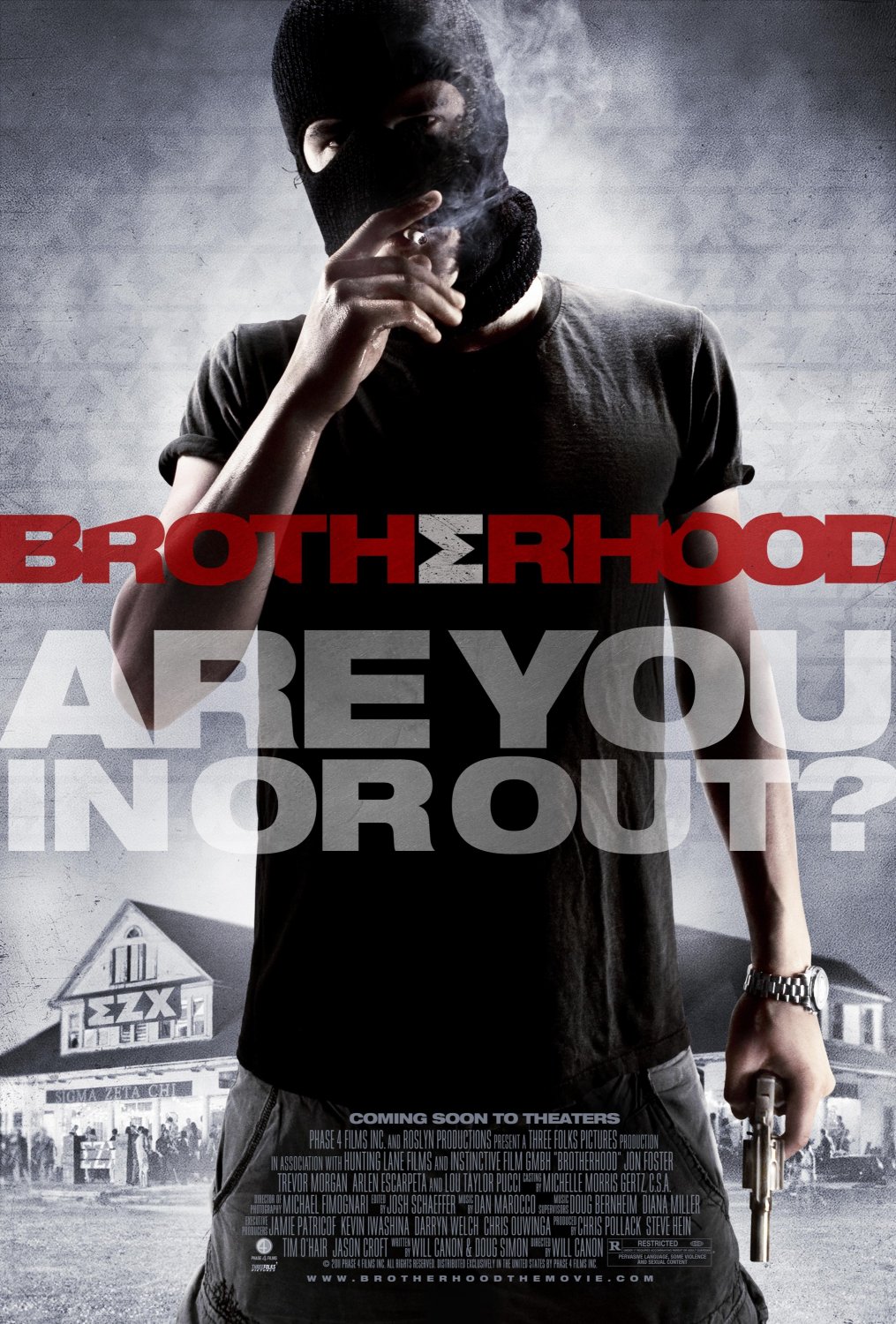A haunting movie poster features a grayscale background with a repeating pattern of sigma and chi Greek letters, hinting at a sinister fraternity theme. Central to the image stands a white male figure, clad in a black t-shirt, black pants, and a black ski mask, revealing only his eyes. With a cigarette held to his mouth by his right hand and a gun pointed downward in his left hand, outfitted with a wristwatch, he exudes an aura of menacing secrecy. Behind him looms a building labeled "EZX," likely a fraternity house, with ominous figures gathered outside, shrouded in shadow. The bold red title "Brotherhood," with an inverted E, dominates the middle of the poster, accompanied by the tagline, "Are You In or Out?" in translucent white text. Below, in small unreadable font, additional credits suggest a forthcoming cinematic release, adding an extra layer of intrigue to the mysterious and foreboding scene.